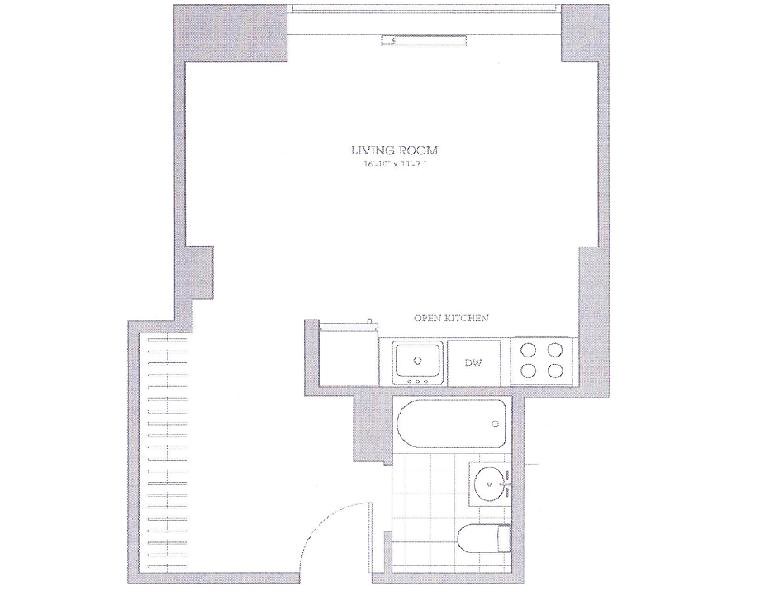This image displays an aerial, bird's-eye view of a minimalistic floor plan in shades of white and gray. At the top of the image, the area labeled "Living Room" is presented in a subtle, faded gray font within a spacious, square region. Directly below the living room, the space transitions into an "Open Kitchen," also labeled in a light gray font. The kitchen layout showcases the rudimentary outlines of essential appliances: a stove, a dishwasher, a sink, and a refrigerator.

Separated by a wall partition, the adjacent area reveals a compact bathroom setup, which includes a bathtub, a small sink, and a toilet, all outlined in gray. On the other side of the floor plan, there's another roughly sketched square section containing a series of gray squares, likely representing furniture or additional fixtures.

The entire floor plan has a slightly pixelated, yet largely clear and legible quality, making it easy to understand the layout and design despite its faded appearance.